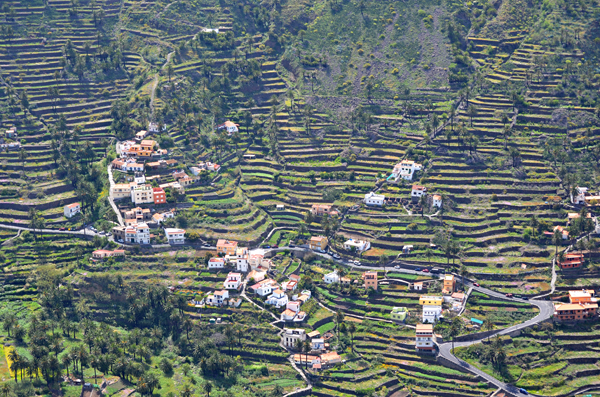The image depicts an expansive aerial view from a high vantage point, possibly from a helicopter, showcasing a picturesque village nestled on the side of a lush, tiered mountainside. The mountainside is adorned with extensive green terraces, resembling large steps, which could potentially be agricultural plots such as rice fields. The scene is vibrant with an array of greens, browns, and occasional hints of blue, indicating various elements like vehicles or canopies scattered throughout.

The village appears predominantly in the lower portion and along the edges of the image. The homes are mostly white with brown roofs, clumped together in small pockets at the left bottom, the right, and the center of the view. The center section of the image is relatively sparse, featuring a few isolated dwellings, while the right center edge displays a more concentrated cluster of buildings.

Tall trees, predominantly green, frame the upper third of the image, creating a canopy over the village. A striking contrast is observed on the right side where trees bear purplish-gray stems and branches, possibly indicative of the onset of winter, as these trees appear to be shedding their leaves.

There is a network of gray asphalt roads weaving through the fields and between the houses, enhancing the image's organized and patterned layout. The terrain is brightly illuminated by natural daylight, giving the photograph a clear and vibrant appearance. No text or numerical data is present in this visually captivating image of a serene and well-planned village landscape.